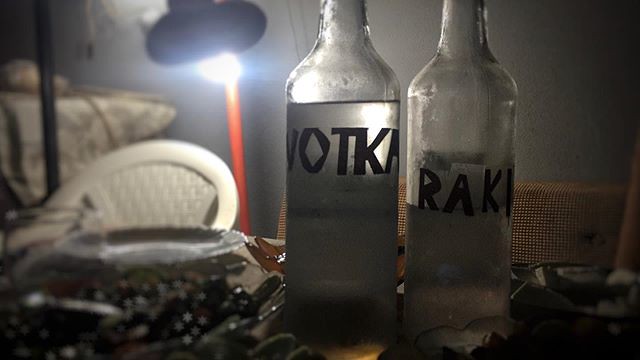The image depicts a somewhat dark room, illuminated by a single red pole light. In the foreground, two clear glass bottles are positioned on a desk. The bottle on the left, nearly filled to the top with a clear liquid, has "VOTKA" scrawled in an odd handwriting. The bottle on the right is half empty, displaying only part of its label, "R-A-K," in a similar black font. Both bottles exhibit signs of condensation. Behind the desk and slightly to the right, there are two high-back chairs with woven wooden seats visible. Directly underneath the light is a white plastic lawn chair. The desk itself holds a few knick-knacks, including a couple of ashtrays, adding to the overall ambiance of the scene.